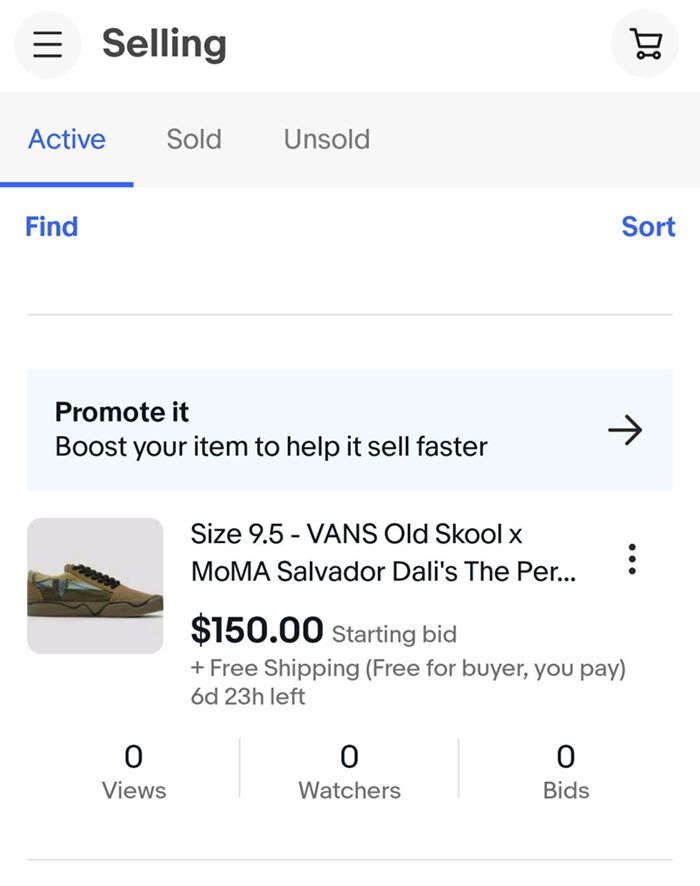Displayed prominently at the top of the screen, numerous options are available: "Selling," "Shopping Cart," "Active," "Sold," "Unsold," "Find," and "Sort." A banner reads "Promoted: Boost your item to help it sell faster" with a right arrow for further action. 

Featured in the forefront is a brown shoe with detailed shoelaces against a gray background. The listing highlights the shoe size as 9.5 with the title "Advanced Old School X MoMA Salvador Dalí Slipper..." The starting bid for the item is set at $150, including free shipping with the note "Free for buyer; you pay." The auction has a duration of six days and 23 hours remaining. 

The current activity status shows no reviews, watchers, or bids. The layout revisits the "Active," "Find," "Sold," "Unsold," "Sort," and "Promoted" options with the prompt to "Boost your item to help it sell faster" against a blue backdrop. The visual features a black woman modeling brown shoes, emphasizing the shoe’s title, "Advanced Old School."